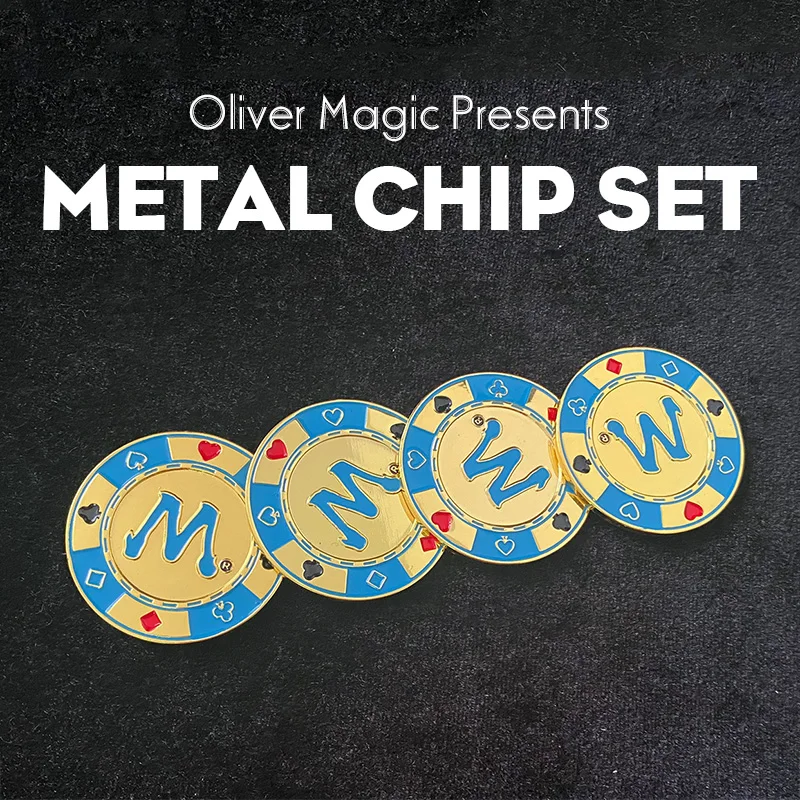The image showcases a promotional poster for "Oliver Magic Presents: Metal Chip Set," set against a sleek black background. Featured prominently are intricately designed metal gambling chips that exude an air of sophistication and luxury. Each chip bears a central "W" in elegant blue text set on a light yellow or tan background, hinting at a possible connection to a brand or a special event.

Surrounding the central emblem on the edge of each chip are detailed depictions of card suits—hearts, diamonds, and spades—meticulously arranged to enhance visual appeal. The hearts are rendered in vivid red against a tan background, while the spades stand out in striking black. Similarly, additional hearts and diamonds appear against a rich blue background, adding contrast and depth to the design.

The metallic surface of the chips suggests a gold or brass finish, lending a sense of opulence to the set. The careful placement of each card suit and the distinct "W" emblem make these chips a unique and eye-catching addition to any collection, underscoring the craftsmanship and attention to detail inherent in their design.